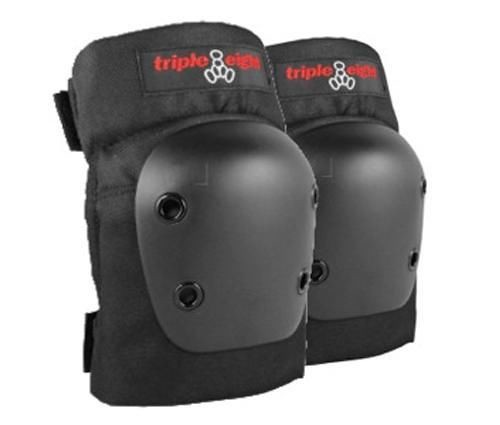This is a detailed product image of a pair of black knee pads, likely sourced from the internet. Each knee pad features a dark gray, hard protective cup on the exterior, designed to shield the knees during activities, suggesting use in sports. The knee pads have Velcro straps at the top and bottom for secure attachment around the leg. Notably, a tag at the top of each pad displays the brand "Triple 8" in red lettering, accompanied by a white circular design that includes two small circles aligned vertically and another pair of circles off to the side, resembling legs. Both knee pads in the image appear identical, although one pad is positioned slightly closer to the viewer, partially obscuring the other.